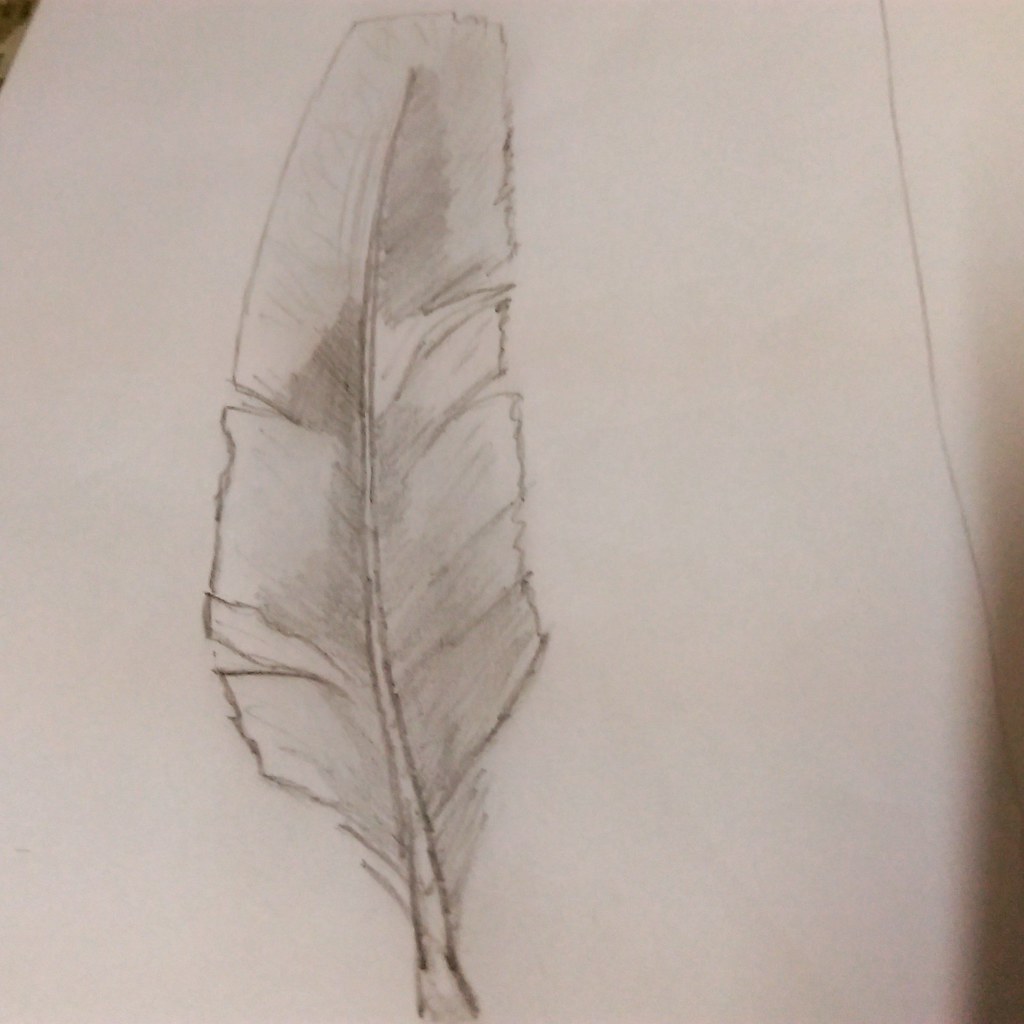This image depicts a detailed pencil sketch of a feather on white paper that appears slightly angled, revealing a bit of the background in the top left corner. The feather, likely drawn with a charcoal or regular pencil, is rendered with intricate details, including subtle indentations that lend it a realistic appearance. The feather has a rounded top, rather than the usual pointed tip, and its stem starts thicker at the base before tapering as it extends into the body of the feather. The sketch is vertically oriented, and there is a long, vertical pencil line to the right, suggesting it may continue off-frame. The feather is meticulously shaded and outlined, capturing the artist's attention to detail. The paper itself is clean with no additional marks or elements besides the feather and the vertical line.